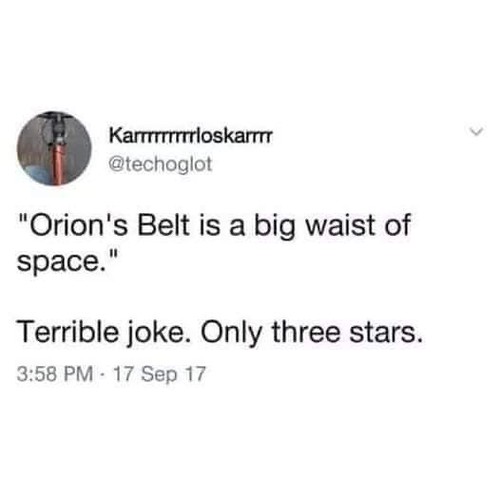A screenshot from social media captures the profile of user CarlOscar, handle @techo-glot, with the display name formatted as K-A-R-R-R-R-R-R-L-O-S-K-A-R-R-R. The profile picture in the upper left corner shows an emblem resembling a bike pump with a black top and pewter handle against a gray background. Below the handle, in black text, the user has humorously shared, "Orion's belt is a big waste of space," with "waste" cleverly misspelled as "waist." An observer wittily responds, "Terrible joke, only three stars." The post is time-stamped at 3:58 PM on September 17, 2017, with a subtle gray down arrow in the upper right corner indicating more options.